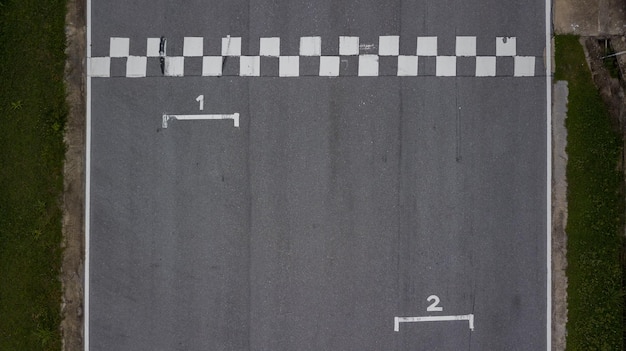This top-view photograph showcases a wide, grey concrete race track that fills most of the frame. The track features prominent white markings, including checkerboard squares forming a line, which likely represents the start and finish line. Positioned near this line are the starting positions marked with the numbers "1" and "2," with position "1" closer to the line and position "2" situated slightly further back. Flanking the track on both sides, lush green grass contrasts vividly with the track's grey surface.